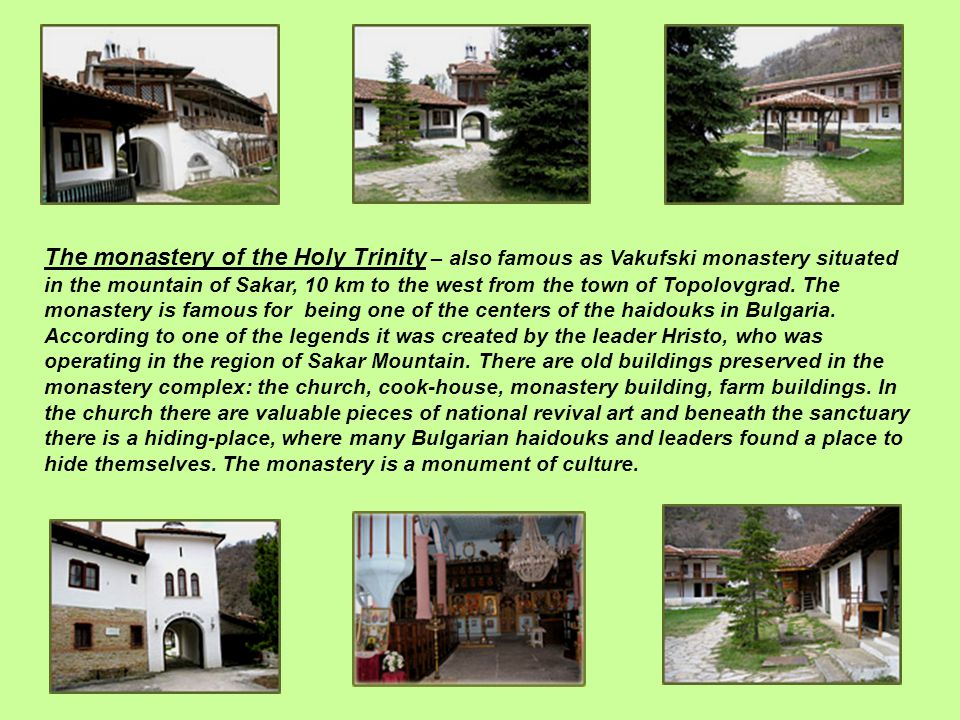The image resembles a slide from an educational PowerPoint presentation with a light green background featuring six small rectangular photographs arranged in two rows—three at the top and three at the bottom. In the middle lies a block of text titled "The Monastery of the Holy Trinity," also known as Vakufsky Monastery. This monastery, located in the Sakhar Mountain 10 kilometers west of Topolovgrad, is one of the famed centers of the High Dukes in Bulgaria. According to legend, it was established by a leader named Hristo. The complex contains several preserved old buildings, including the church, cookhouse, monastery building, and farm structures. The church houses valuable pieces of National Revival art and beneath the sanctuary lies a hiding place historically used by Bulgarian High Dukes and leaders. The top left photo shows part of a building with an arched passageway, while the top middle captures a paved path and trees in a courtyard. The top right image features a gazebo with surrounding greenery. The bottom left showcases another monastery building, and the bottom middle displays the ornate, Eastern European styled interior with gilded decorations and a chandelier. The bottom right photo presents an outdoor scene with stone paths, grass, trees, and enclosing buildings. The monastery is recognized as a cultural monument.